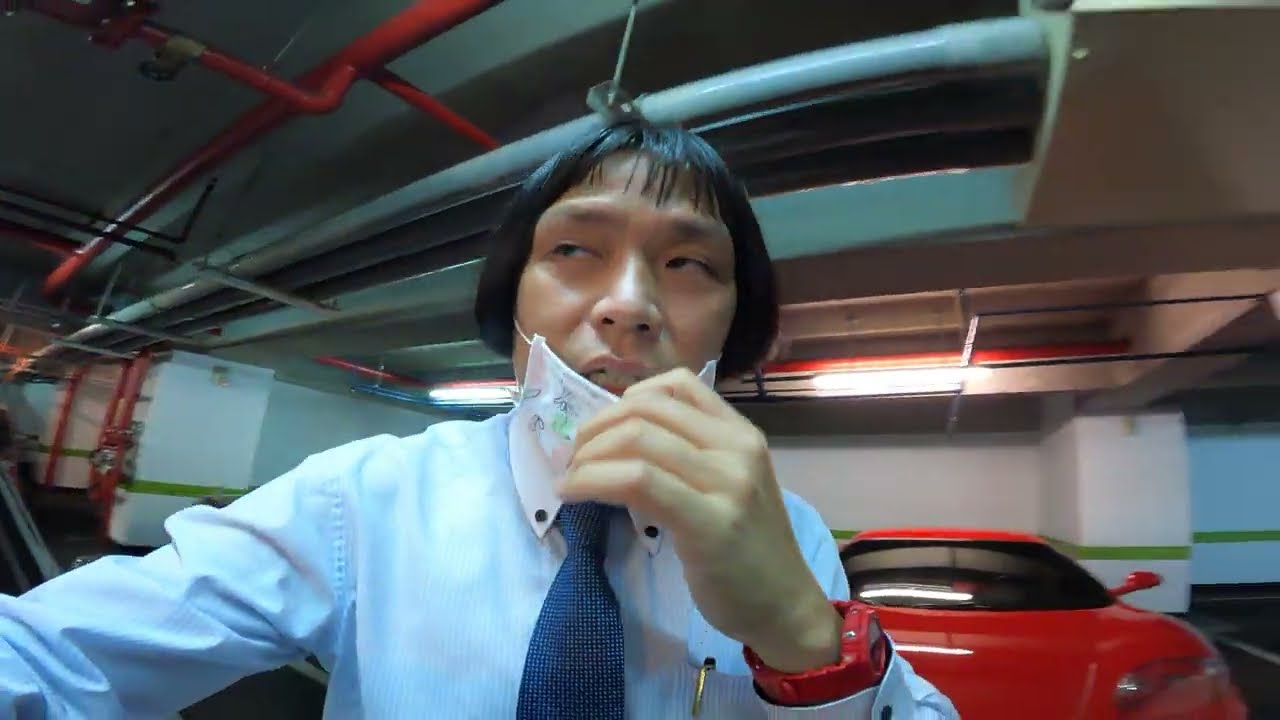In an indoor parking garage, an adult male with shoulder-length black hair and Asian features is captured in a photograph standing centrally while looking to the left. He is pulling down a white cloth face mask with his left hand, partially revealing his mouth and nose. He is dressed in a button-up blue shirt with a white collar, complemented by a white and blue checkered tie. His left breast pocket contains a gold and black pen, while his left wrist sports a prominent red wristwatch. The backdrop includes a sleek two-door red sports car, parked against a white wall adorned with a green stripe running horizontally along the bottom. Above him, gray and white pipes crisscross the ceiling, adding to the industrial ambiance of the parking facility.